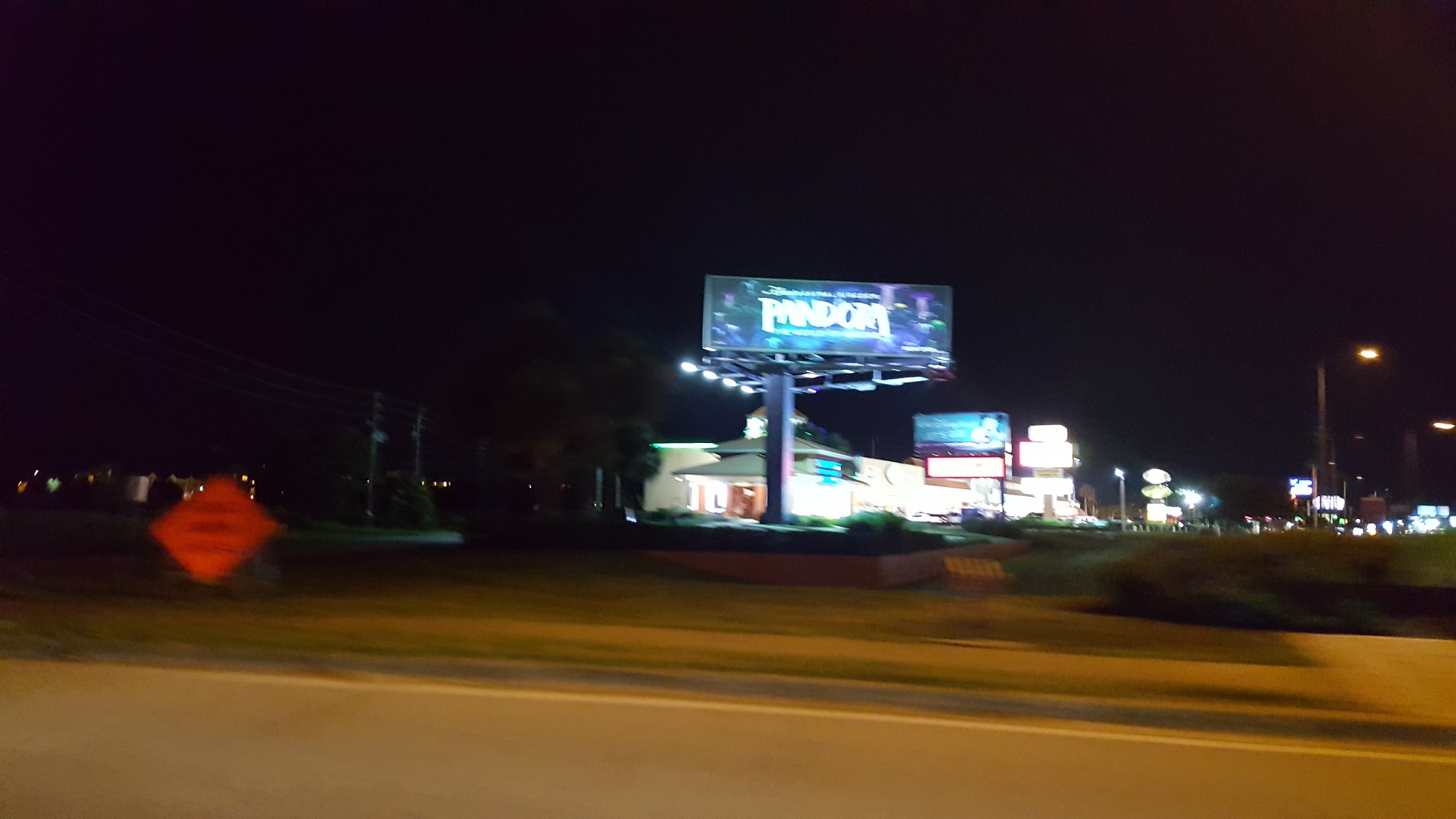This nighttime photograph, likely taken from a moving vehicle with the window rolled down, captures a bustling urban scene. Prominently featured in the foreground is an orange, diamond-shaped sign indicating "Road Work Ahead," positioned near a sidewalk lined with grass strips and bushes. Several light poles illuminate the area, adding to the urban ambiance. Multiple business signs in the background signal an active and open commercial district, possibly a strip mall. Vehicles are visible on the road, contributing to the sense of movement and activity. The dark sky overhead contrasts sharply with the artificial lights below. A striking black and purple billboard with white lettering—including the word "Fandom," which suggests it advertises a nearby restaurant or store—looms in the background. The overall scene evokes the lively atmosphere of a city at night, with various elements hinting at ongoing road maintenance and the presence of numerous businesses.